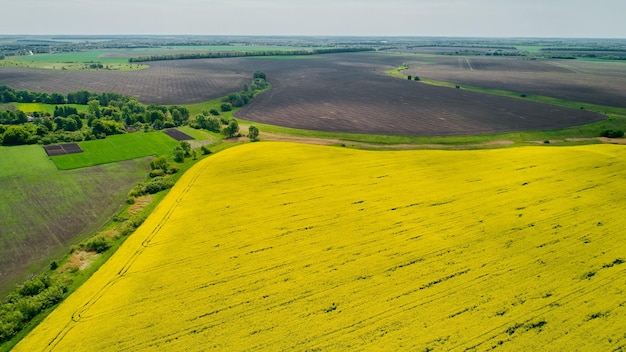This aerial photograph captures a vast farming landscape with a diverse palette of colors and terrains. The fields are clearly delineated in geometrically even patches, showcasing a range of agricultural textures and hues. The largest areas are a striking golden yellow, suggesting a mature and possibly flowering crop, while other sections display a robust green vegetation, interspersed with some tilled brown soil. There's also a notable section of purple-hued fields adding a unique vibrancy to the scene. Shrubs and trees pepper the landscape, particularly to the left, contributing to the lush greenery. The terrain is mostly flat, with the horizon marked by a subtle gray, overcast sky, indicating a cloudy day. The distant horizon is lined with dense trees, and shadows of clouds can be discerned on the ground below, highlighting the mix of light and shadow across the fields. Bright sunlight reflects off parts of the terrain, adding a dynamic contrast to the scene. The image, taken during daytime, beautifully encapsulates the varying elements of this fertile and meticulously parceled farming area.